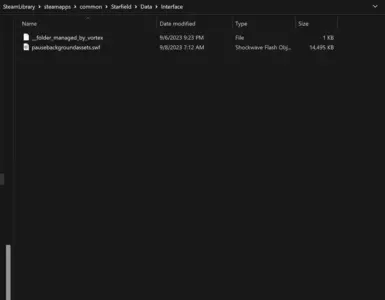The image showcases a File Explorer window displaying the contents of a directory. The items within this directory are organized in alphabetical order. The path to this directory is clearly visible and reads: "STEAM library > STEAMapps > common > Starfield > Data > Interface." Notably, this folder is managed by Vortex. The interface features a black background with white text for clear readability. Two files are present in the directory: the first file is 1 KB in size, while the second file is significantly larger, measuring 14,495 KB.